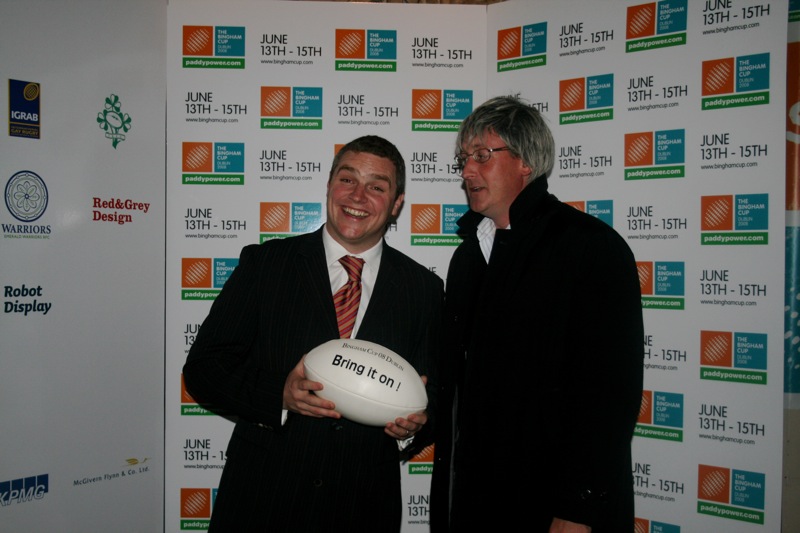In a color photograph with a landscape orientation, two gentlemen are prominently standing in front of a Step and Repeat backdrop, promoting an event scheduled from June 13th to June 15th. The backdrop features multiple indistinct square logos in orange and blue. To the left are sponsor logos, notably from KPMG, Red and Gray Design, and Robot Display. The younger man on the left is in a black suit with a white shirt and red tie, smiling and holding a white football emblazoned with the phrase "Bring it on" in black text. Beside him, an older man with salt and pepper hair, glasses, and a black overcoat, is smiling while looking at the football. The image captures a moment of camaraderie at what appears to be a professionally significant event.